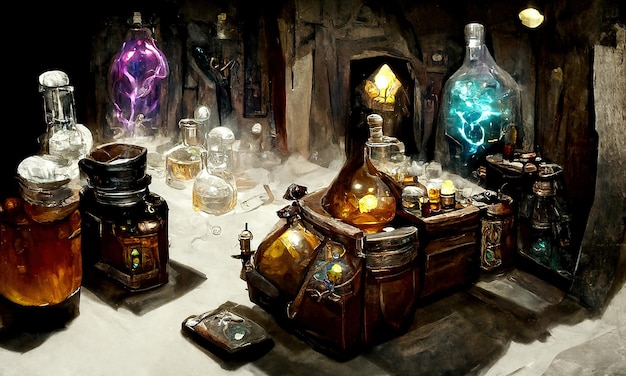The image depicts a mystical, dark setting resembling an alchemist's table or a witch's workbench, painted in a detailed, oil painting style. At the forefront, a leather bag brimming with assorted bottles takes center stage. The bottles vary from small and rounded to larger, more substantial ones, and contain liquids of various colors, adding to the enigmatic ambiance. To the right of the leather bag, a prominent bottle filled with a bright, glowing blue substance stands out. There is also a book placed to the left of the bag. Further to the right, a container holds numerous transparent and colored bottles, enhancing the scene's complexity.

To the left side of the composition, three large jugs are noticeable, one with an amber hue and another containing a green substance. Behind these jugs, there are two more significant bottles illuminated by purple and aqua blue lights, contributing to the scene's magical aura. The background is predominantly dark, save for an opening that reveals a hint of yellow light, adding to the mysterious and mystical feel. This artistic creation skillfully combines elements of witchcraft and alchemy, evoking an atmosphere ripe for spellcasting and potion-making.